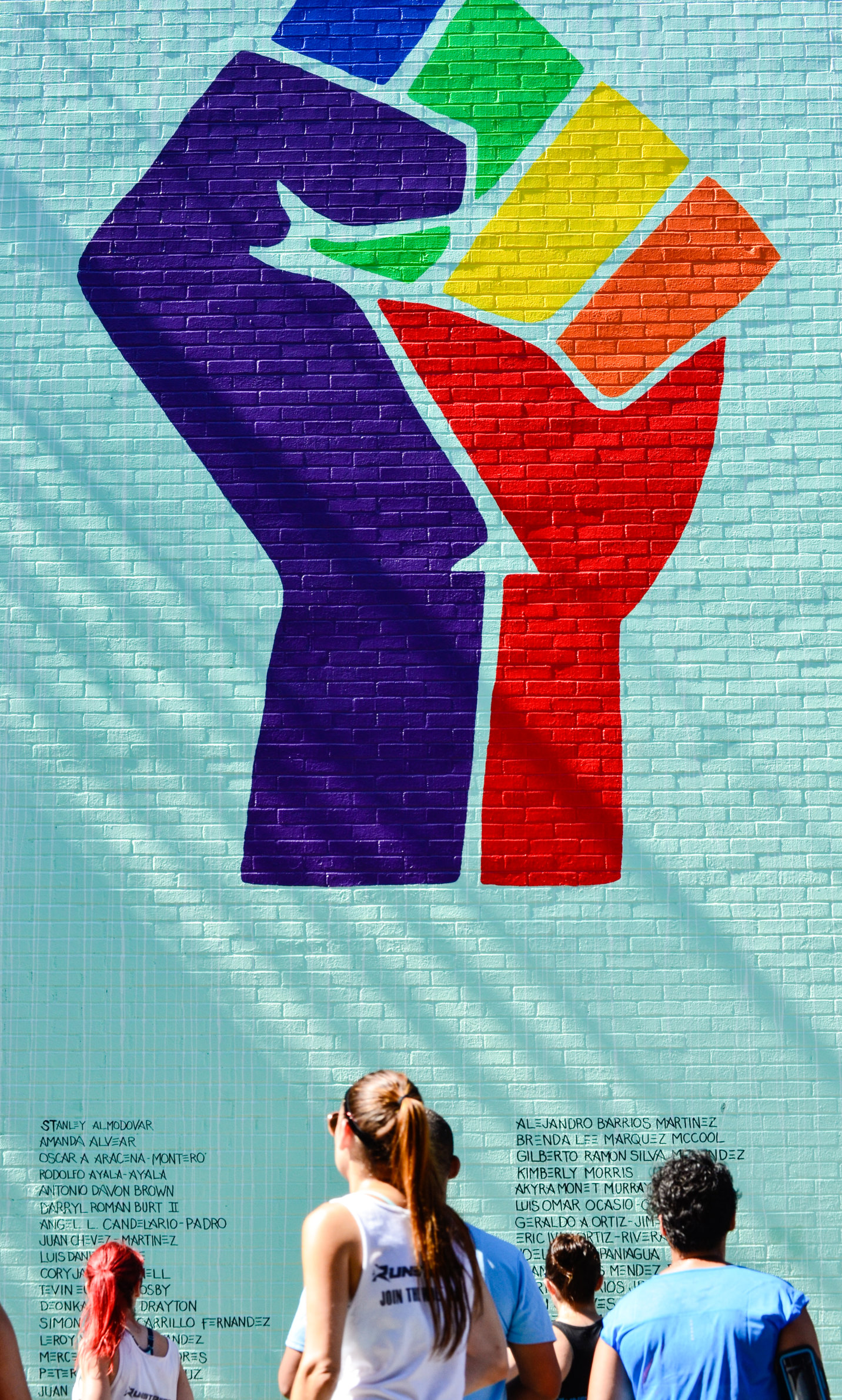The image depicts a light powder blue brick wall with a large, vibrant mural of a clenched fist, symbolizing power and solidarity, often associated with the Black Lives Matter movement. The fist is vividly colored: the thumb is purple, the index finger is blue, the middle finger is green, the ring finger is yellow, the pinky is orange, and the side of the palm is red. A white arrow starts at the wrist and extends diagonally upwards towards the hand. Below the fist are names, suggesting this may be a memorial wall. Six onlookers stand before the mural, their backs to the camera, seemingly admiring the artwork. Notably, two women have long ponytails—one brunette and one redhead.